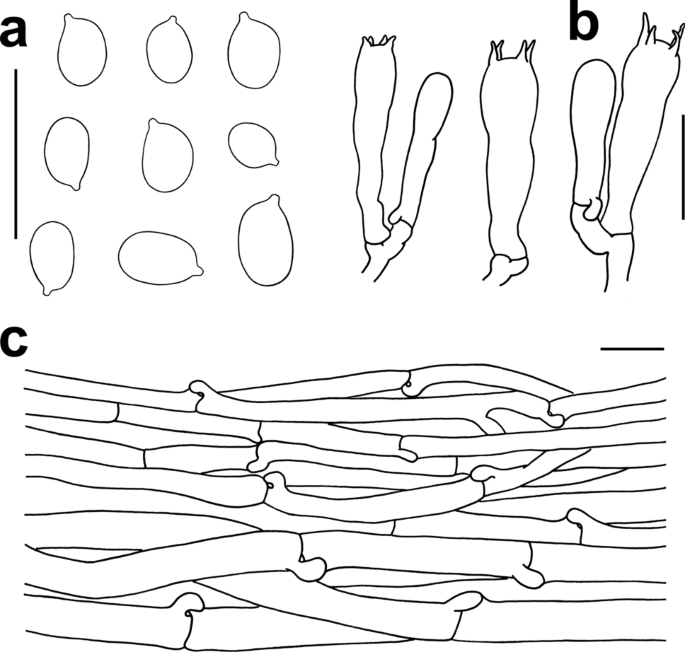This is a highly detailed, black-and-white illustration that seems to be a stylized, pen-and-ink drawing, potentially hand-drawn or computer-simulated to mimic a hand-drawn effect. The image is organized into three distinct sections, labeled A, B, and C, and arranged within a square format.

In the top left quadrant (section A), there are nine oval objects with dark outlines and white centers, organized in a 3x3 grid pattern. These objects resemble seeds or lemon shapes and are next to a bold, lowercase "a."

Moving to the top right quadrant (section B), the illustration depicts three bulbous forms or possibly unbloomed plant buds. Two of these forms are paired together, while the third stands alone. Small tendrils or spikes emerge from the tops of these shapes, and a bold, lowercase "b" is placed next to them.

The entire bottom portion of the image (section C) displays a broader, interconnected series of stems or sticks, linked together in sections. This horizontal assembly of forms suggests a complex structure, resembling either botanical stems or elongated bones. This section is labeled with a bold, lowercase "c."

Overall, the image gives an impression of an intricate, botanical or anatomical study rendered in a minimalist, black-and-white style.